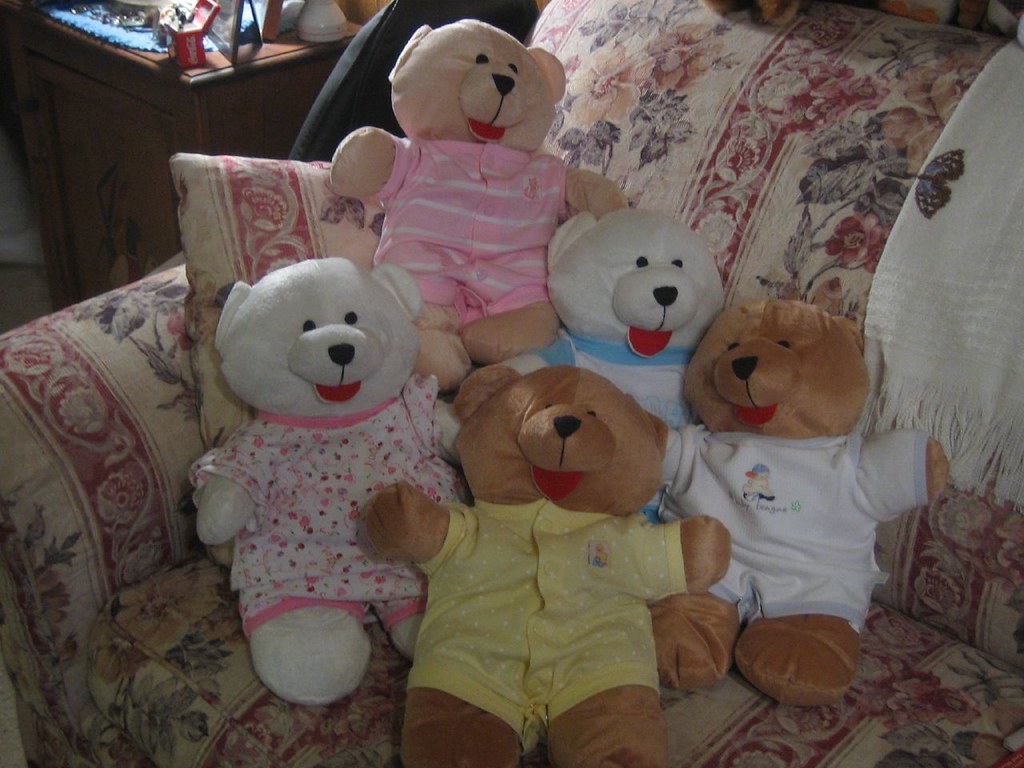This indoor photograph showcases a cozy living room scene featuring a wooden cabinet adorned with various knickknacks and a lamp, providing ambient lighting. The main focus, however, is a beige couch with an intricate floral embroidery design in vibrant hues of red, orange, purple, and blue flowers, combined with white and maroon leaves and square patterns. Draped over the back of the couch is a pillow and blanket.

Seated prominently on the couch are five adorable teddy bears, each with unique characteristics. Starting from the left, there's a tan bear sporting a pink shirt with white stripes. Beside it, a white bear wears a white shirt with pink rims and tiny dotted designs, possibly resembling small fruits. Next is a brown bear adorned in a yellow outfit dotted with white polka dots, followed by another brown bear in a white shirt featuring a graphic that looks like a duck riding a vehicle. Finally, on the right, there's a white bear in a white shirt with a blue border. All of these teddy bears share a common feature - they have their tongues sticking out, adding a whimsical touch to the scene.